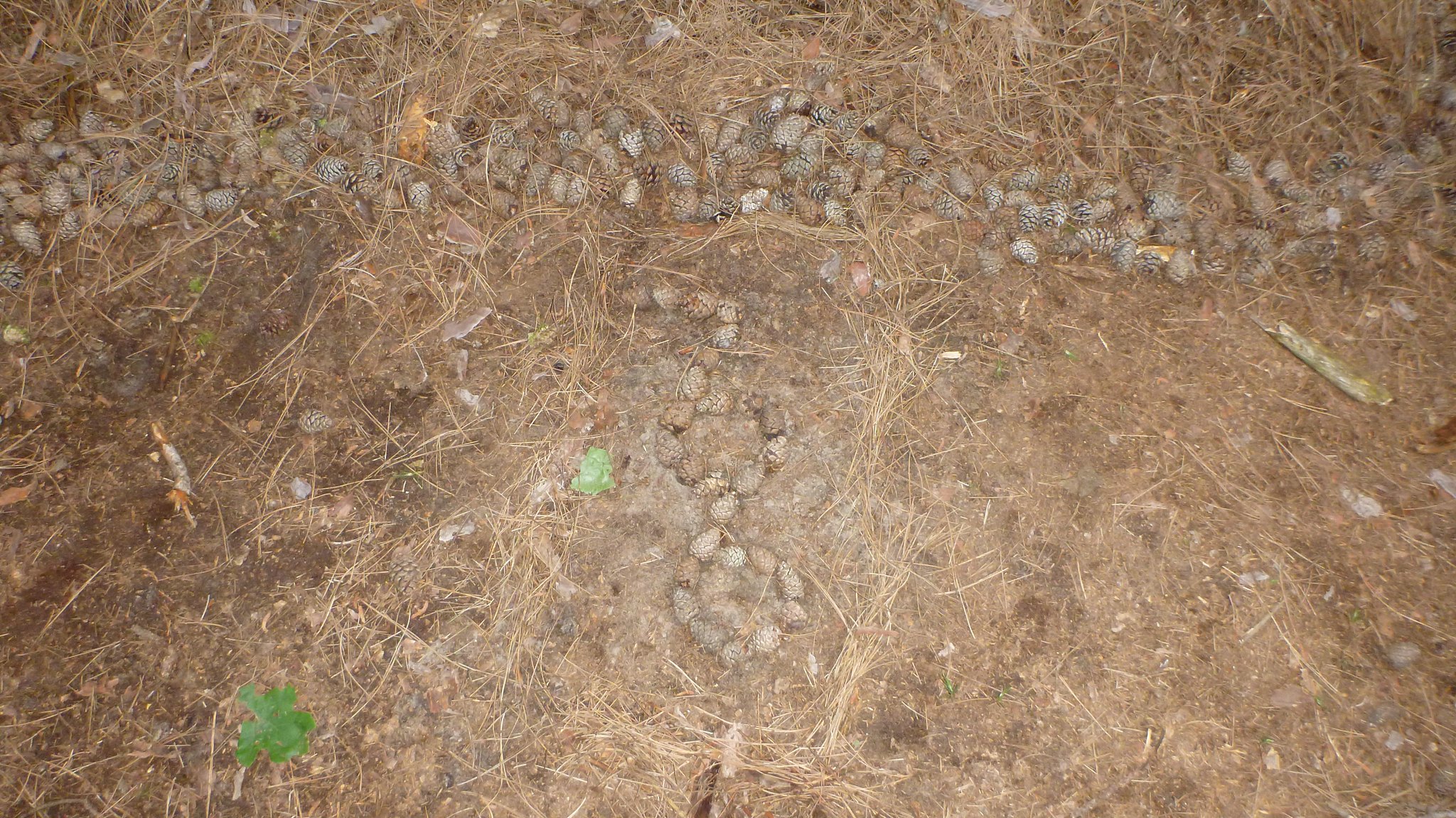The photograph, taken from an overhead perspective, primarily showcases a large patch of bare brown dirt intermixed with areas of dead, brown grass and scattered hay. The ground features sparse green sprouts emerging here and there. At the top of the image, stretching from left to right, there's a pathway composed of gray pine cones and rocks arranged to appear like a makeshift rock wall. This pathway, adorned with dry grass and sticks, creates a noticeable border. Centrally located within the dirt expanse and framed by dry grass, there's a distinct design made from the rocks and pine cones: an arrow pointing right at the top, followed by two zeros stacked vertically below it. This intricate pattern somewhat resembles a figure eight, adding an element of intentional artistry to the otherwise barren ground.